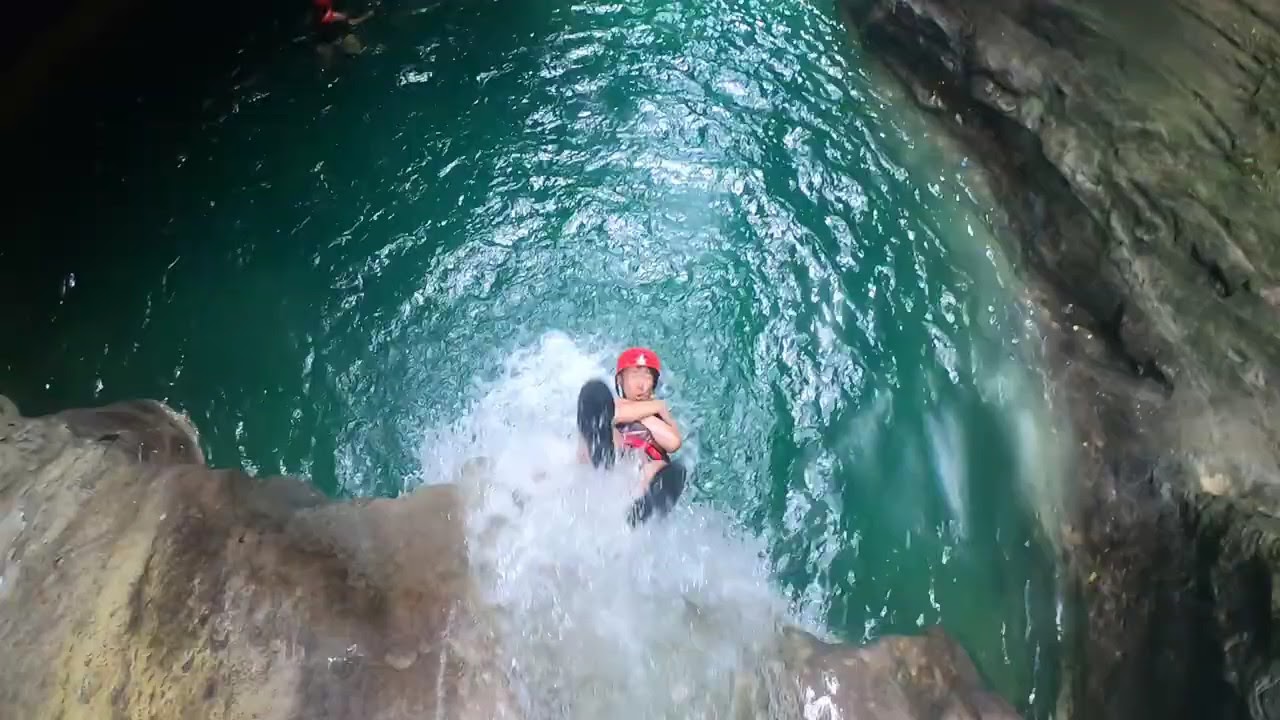In a breathtaking outdoor photograph taken during the daytime, a brave man of Asian descent is captured mid-dive as he descends backward from a steep, tan, and yellow-colored cliff into a stunning, emerald-green natural pool below. Equipped with black water shoes, a red helmet, a life vest, and gray swim shorts, the diver's eyes are closed, and his arms are crossed over his chest, highlighting the intensity of the moment. The rocky cliff face, smooth at the top, slants downward with a powerful waterfall cascading into the pool. In the top left corner of the image, another person, wearing a black swimsuit and an orange life vest, floats serenely in the clear green waters, adding depth and context to the adventurous scene. The steep rock facings framing the pool and the dynamic water currents complete the dramatic and picturesque setting.